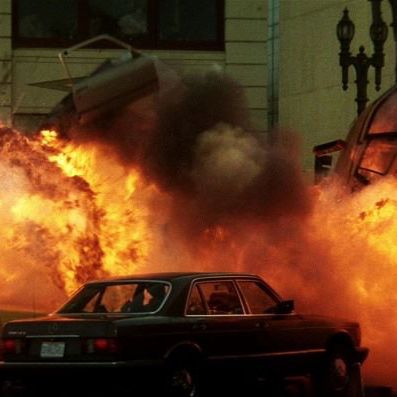In this detailed photograph, we see a dramatic explosion occurring in an urban setting, centered around a mid-1990s, dark-colored, squarish car. The intense burst of fire features bright oranges and yellows, with thick black and gray smoke rising above it. A car door, gray in color, is propelled into the air to the top left of the image. To the right, a black lamppost stands visible against the chaos. Behind the explosion, a greenish-brownish building wraps around the scene, incorporating a wide, black-topped window. The car, positioned centrally, has red taillights, a white license plate, and partially visible interior showing a passenger seat, possibly with an occupant. Another object, perhaps a long, light brown or gray car, is in the foreground with people inside, seemingly driving into the inferno. The detailed background and structural elements emphasize the surreal and violent nature of the moment captured.